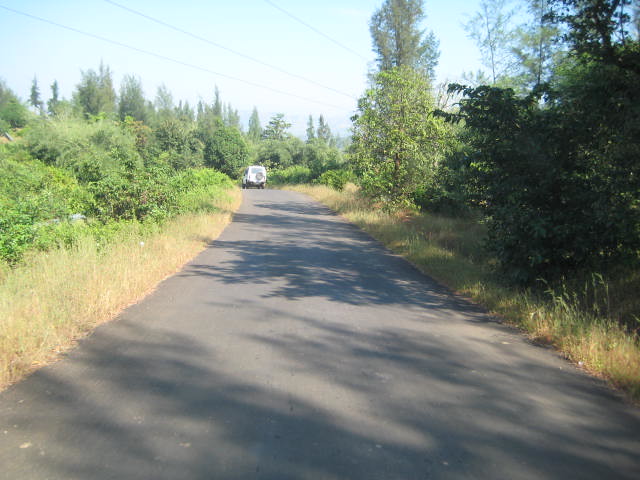A winding black gravel road extends through a natural area with an abundance of small trees, bushes, and tall dead grass flanking both sides. The road is devoid of markings and is illuminated by the bright afternoon sun, casting defined shadows of the surrounding vegetation. A white SUV or Jeep with a large spare tire affixed to its rear is positioned on a slight hill at the distant end of the road, heading upwards. Notably, on the top left part of the image, three power lines traverse above the lush greenery. The sky is a clear blue, without a trace of clouds, emphasizing the vibrant yet rugged landscape.